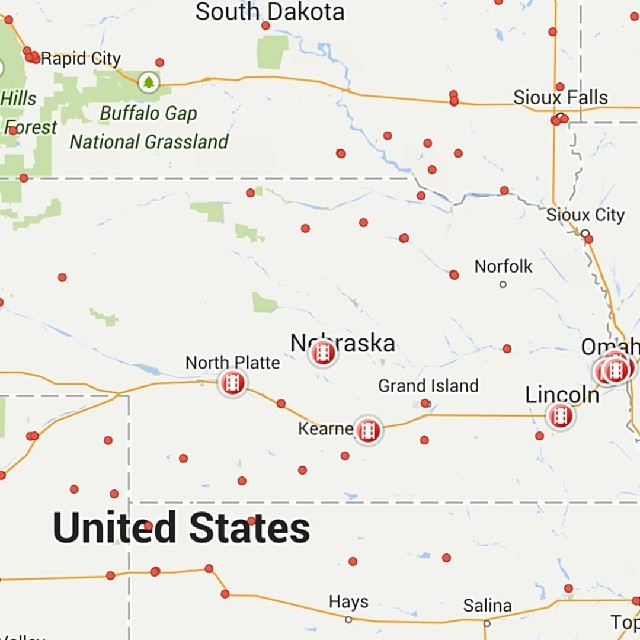Close-up image of a map of the United States, focusing specifically on the state of South Dakota. The map features a white background with yellow lines indicating highways. Scattered throughout the map are red dots marking places of interest, and red circles bordered in white with a white film strip symbolizing movie theaters. In the lower left-hand corner, the map is labeled "United States" in black text. 

At the center top, "South Dakota" is prominently displayed, with various cities and landmarks listed throughout the map. On the left side, "Rapid City" and "Hills Forest" are noted. To the right, "Buffalo Gap National Grassland" can be found. In the upper right section, "Sioux Falls" is marked, with "Sioux City," "Norfolk," "Omaha," "Lincoln," and "Nebraska" listed below it. Further down, additional locations such as "Green Island," "Carnet," "North Plate," "TLP," "Salina," and "Hayes" are indicated in succession.